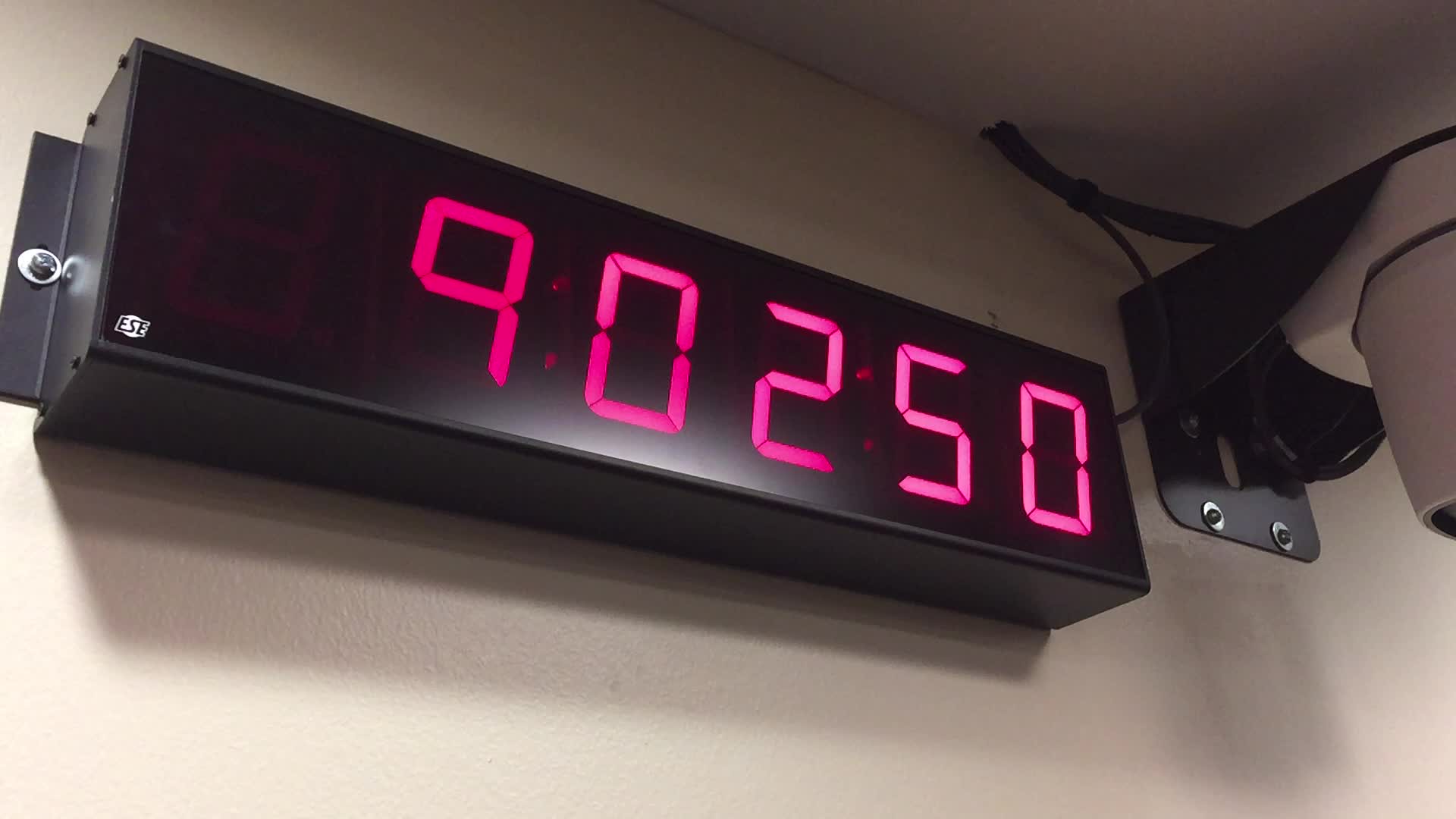The image displays a sleek, modern digital clock mounted high on an eggshell-colored wall. The clock is housed in a rectangular black box, and the time is indicated with bright red digital numbers, which read 9:02:50. This suggests that the seconds are actively being tracked. In the upper right corner of the image, there is an unidentified black bracing structure, secured with two bolts at its base. A visible cable extends from the clock and runs up toward the ceiling. Adjacent to the bracing structure is another indistinct object that is not clearly identifiable from the provided view.